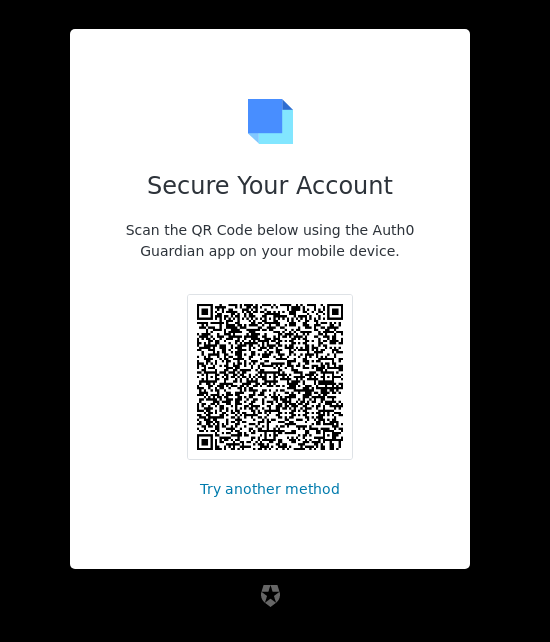The image displays a notification pop-up on a mobile device, prompting users to secure their accounts using the AuthorGuardian app. At the top of the notification, there is a 3D cube icon colored in shades of blue and light blue, with the darker blue facing forward and the lighter blue at the back. Below the icon, the text "Secure Your Account" is prominently featured as the title. Directly beneath this, there is a message instructing users to scan the QR code using the AuthorGuardian app on their mobile devices. The central element of the notice is a square-shaped QR code, consisting of a pattern of black and white squares. Below the QR code, there is an alternative option presented in light blue text, stating "Try another method." The entire notification is bordered by a thick, black frame, adding emphasis to the information within. The pop-up is clearly related to an authentication process for securing the app.